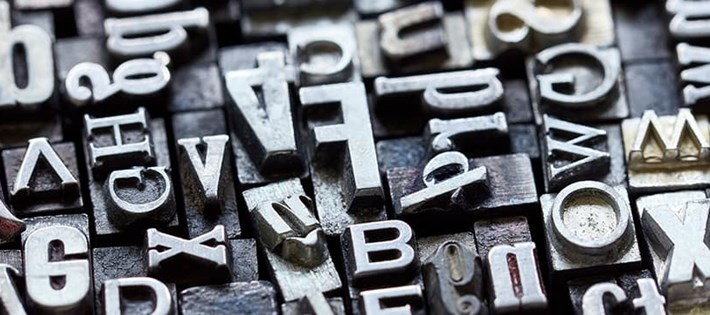This rectangular image, over twice as wide as it is tall, showcases an assortment of printing press letters that resemble stamps. These letters and numbers are set against a dark, almost slate-like, background. The individual blocks, which are either gold or silver, feature extruded, beveled letters on their surfaces. Scattered without any specific pattern, the stamps lie in various orientations—some horizontal, some vertical, some upside down, and others sideways—creating a somewhat messy yet intriguing array. Among the array of characters, one can discern a mix of uppercase and lowercase letters, such as V, H, G, B, P, O, W, and numerals like the number four. The stamps, with their thick and embossed (embezzled) designs, appear to have been used for printing, evoking an old-world charm reminiscent of early printing press techniques.